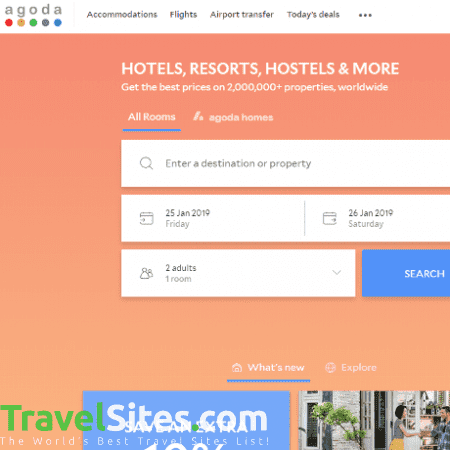This image is a cropped screenshot of a website, specifically from the travel booking platform Agoda. The screenshot captures a square portion of the site, cutting off some content on the right-hand side. At the top of the image, there is a white navigation bar featuring the Agoda logo in grey font, accompanied by five multicolored dots underneath it. Next to the logo, in black font, are several menu options: "Accommodations," "Flights," "Airport Transfers," "Today's Deals," and a menu represented by three black dots.

The background just below the navigation bar is a salmon pink color. Prominently displayed at the top of this section, in white font, are the words "Hotels, Resorts, Hostels, and More. Get the Best Prices on 2 Million+ Properties Worldwide." Directly under this text is a menu where users can choose between "All Rooms" and "Agoda Homes." In the screenshot, the "All Rooms" option has been selected.

Beneath this menu are fields where users can enter search criteria: a destination or property name at the top, followed by check-in and check-out dates, and the number of adults and rooms. Adjacent to these fields is a blue search button. Further down, there is another segment with the headings "What's New" and "Explore" in white font. The "What's New" option is selected as indicated by a blue underline.